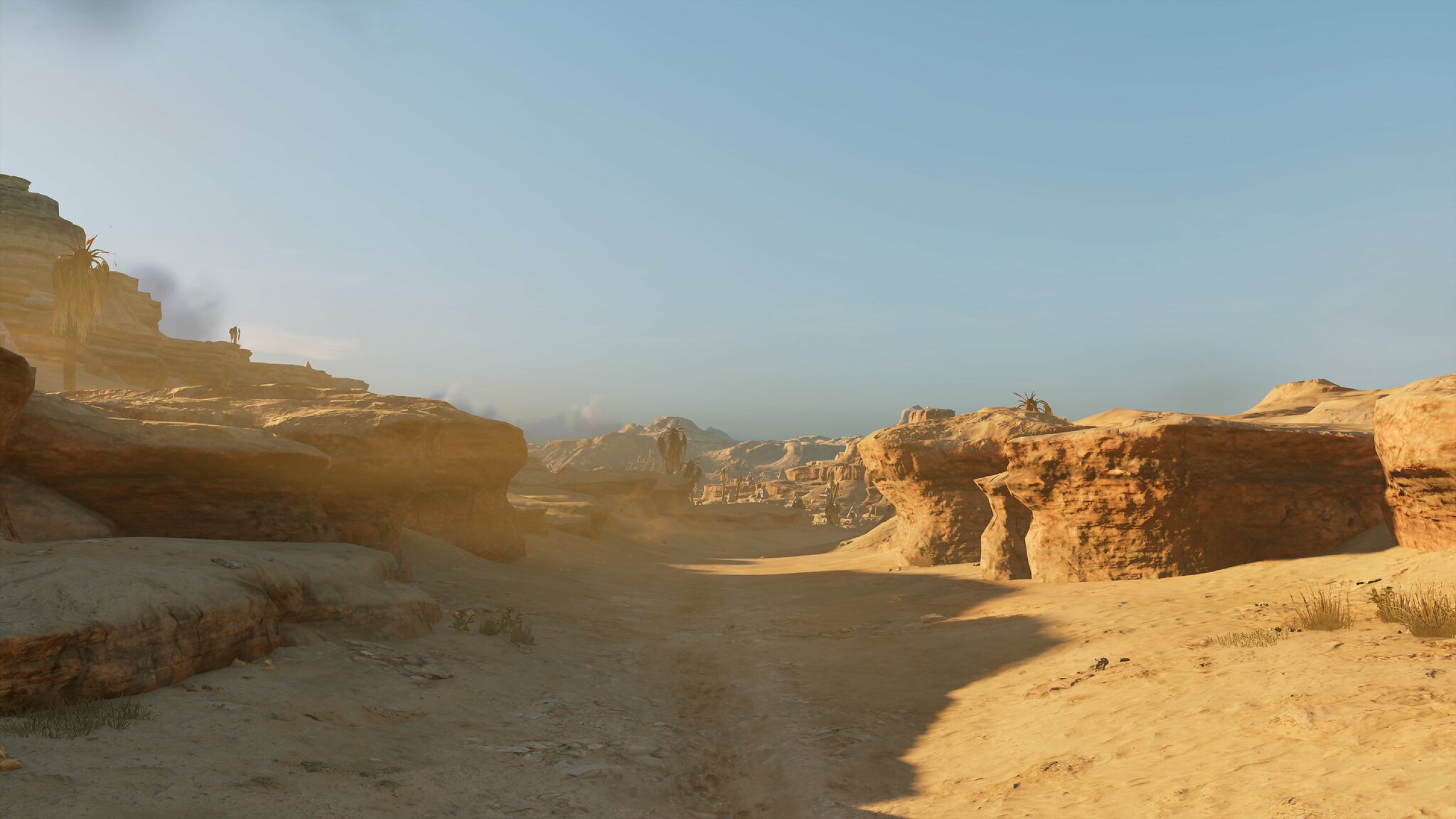A desolate desert landscape stretches across the image, characterized by its dry, sandy or light dirt terrain. The sky overhead is a bluish-gray hue, with only a hint of possible clouds lingering faintly on the left side of the background. Sunlight bathes the right half of the image, casting a warm glow on the ground and the structures, while the left side remains enveloped in shade. Prominently on the right, a cluster of short, biscuit-shaped formations rise up mid-frame, their textured surfaces adding depth to the barren scene. In contrast, taller structures emerge in the shaded background on the left, though they don't reach the top of the frame. The horizon is obscured with indistinct silhouettes, making it difficult to discern whether they are mountains, land formations, or possibly distant townscapes, adding a sense of mystery to the arid expanse.